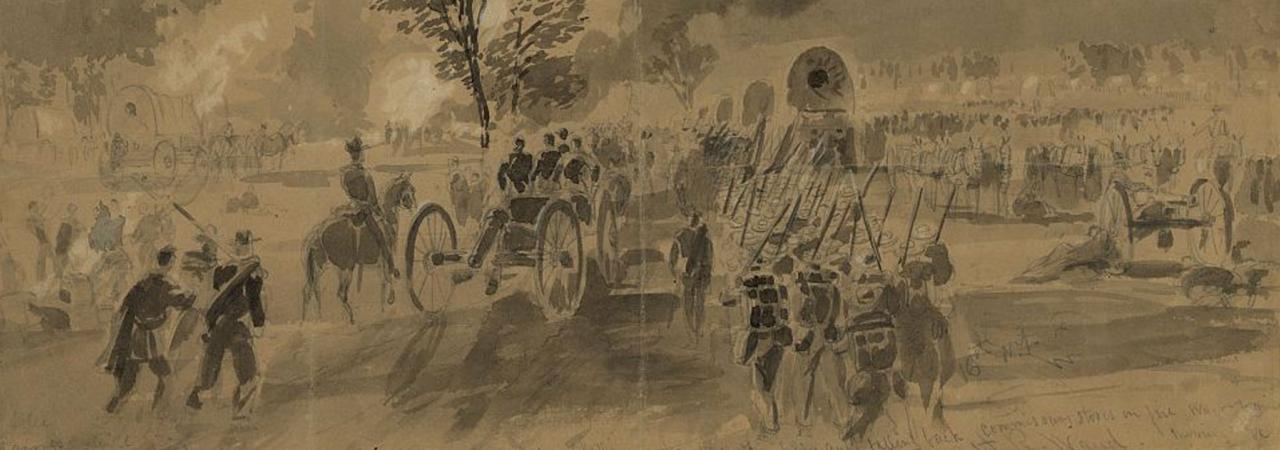The image is a vintage sketch or drawing depicting a wartime scene from the 1800s, rendered in shades of brown, beige, and black. The foreground prominently features a group of soldiers carrying bayonets and long rifles, likely muskets, and wearing backpacks. Some soldiers are on foot while others are on horseback. The figures are drawn in darker shades, which starkly contrast against the brown-toned background. Additionally, there are cannon-like weapons, possibly muskets on wheels, present in the scene. 

In the middle ground, to the left, more soldiers can be seen marching, and there are covered wagons adding to the battlefield atmosphere. The background is less detailed, containing simplified silhouettes of many more soldiers, creating a sense of a vast army moving in the same direction. The composition is accented by a skinny tree with a few leaves in the central background, amidst other indistinct vegetation. Overall, the image captures the essence of a historical battle scene with a multitude of characters and elements contributing to its rich, antiquated aesthetic.